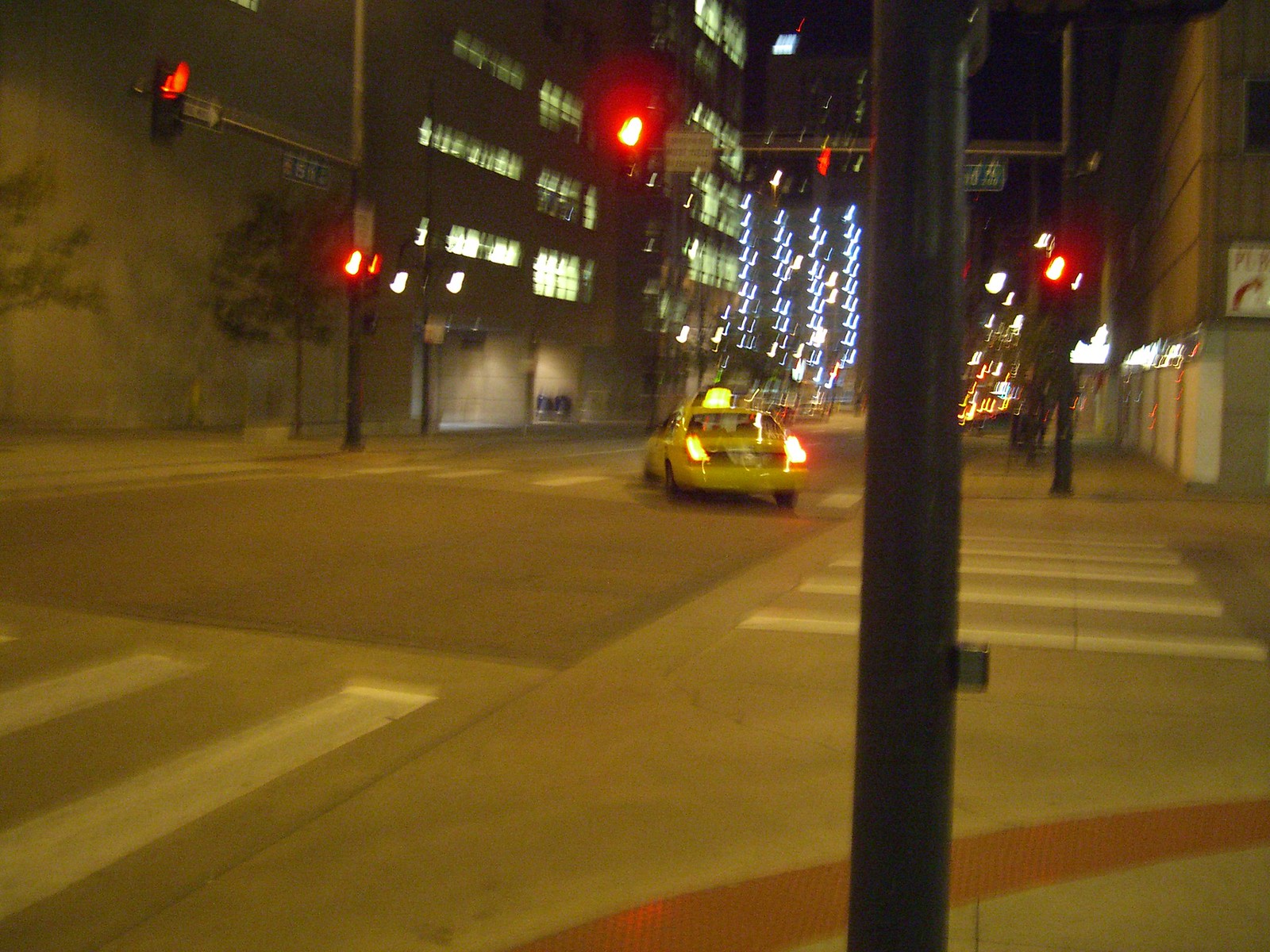This is a blurry photograph of a city street intersection at night, captured under low lighting conditions. The image shows three roads converging, each marked with painted red and white pedestrian crossings, all devoid of people. A yellow taxi with its rooftop taxi sign illuminated and rear lights on is turning onto one of the streets. The traffic lights at the intersection are red. The street is lined with multi-story buildings whose windows are aglow with light, creating a streaky pattern due to the camera's motion. A green street sign is also partially visible, adding to the urban setting.